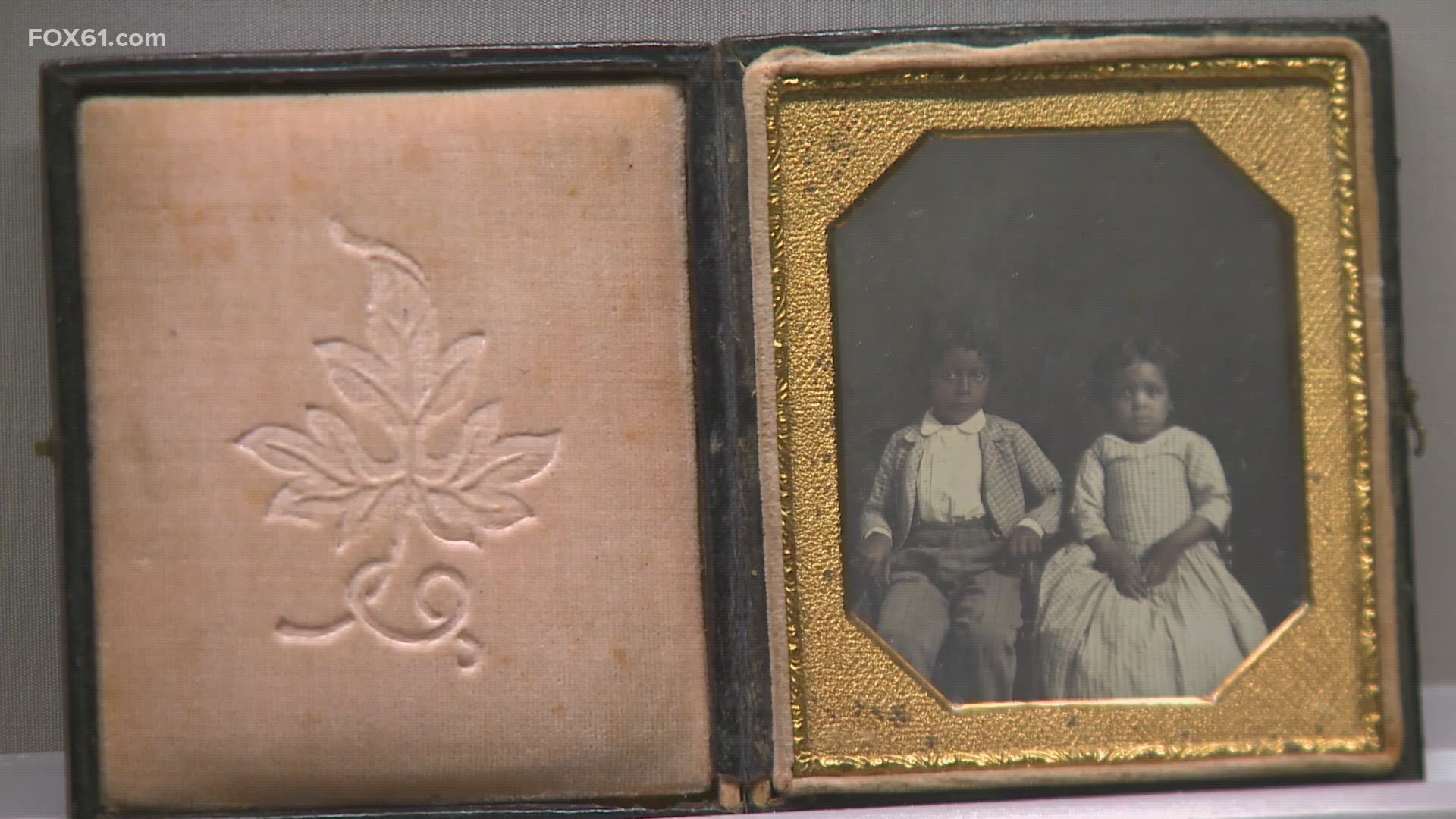The image is a detailed black and white digital photograph framed in a gold, bronze-colored frame. Within the large frame, there are two children: a boy and a girl. The boy, dressed in a white button-up shirt with a light gray jacket and dark gray pants, sits next to the girl, who wears a light-colored, possibly white gown with her hands folded in her lap. Additionally, on the left side of the image, there is another smaller frame with a light pink color, featuring what seems to be a picture or stone with a leaf insignia. The composition and contrast of the elements create a visually compelling scene.